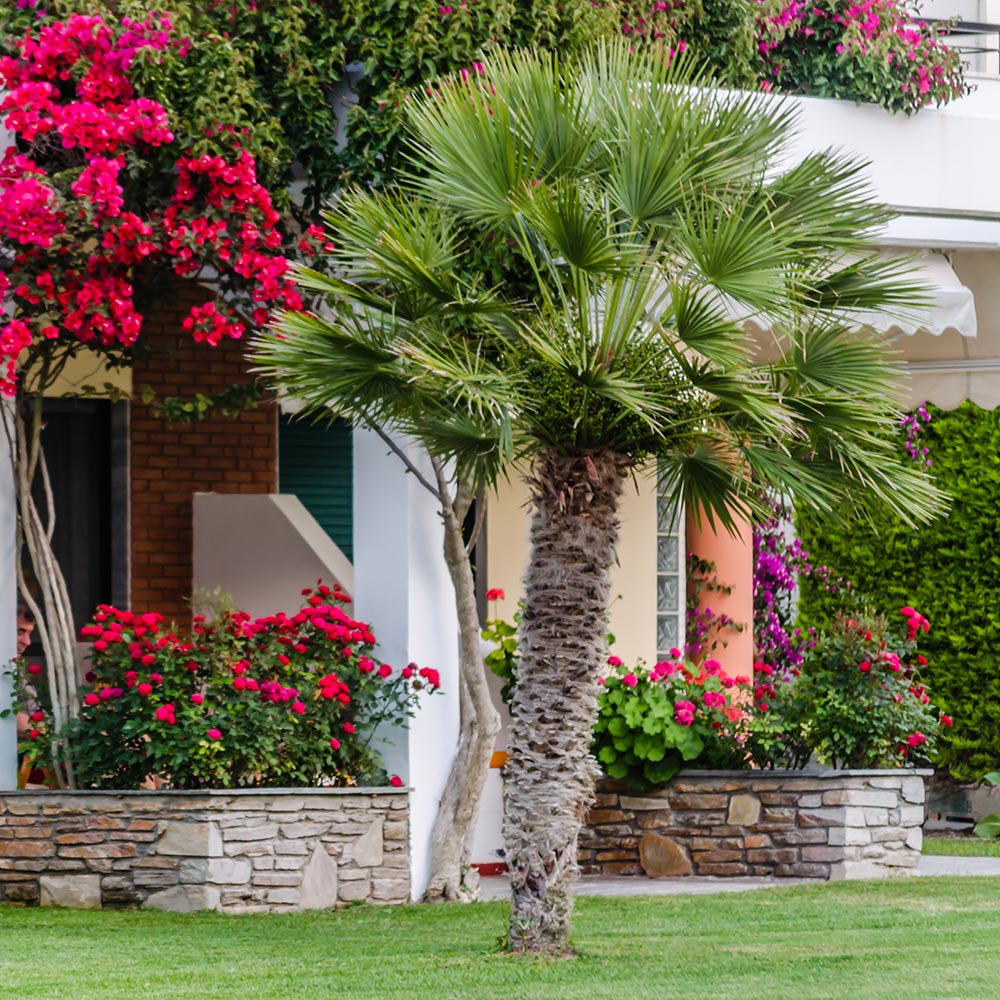This full-color, vertically rectangular photograph captures the front yard of a house taken outdoors during daytime under natural light. Dominating the image is a centrally positioned palm tree with a lean, spiky trunk in shades of light brown and gray, leading up to a crown of green, spiky fronds. Below the tree, the foreground showcases a well-maintained, lush green lawn.

On either side of the palm tree are brick planters. The right planter contains vibrant red and purple flowers, while the left planter features red flowers and a blooming tree with red blossoms. Further back in the scene, to the top left, there is a rose bush with red roses interspersed among green leaves. The house itself, partially visible, features a dark red brick facade with a window or possible sliding glass door mostly obscured by the foliage. A white entryway is noticeable at the top center of the image, with plants climbing along its roof area. Additionally, a pillar is seen in the background on the right, colored in a peachy hue, while a white stairway with a brick wall is also partially visible. The overall impression is one of meticulously tended landscaping with a variety of vibrant blooms framing the central palm tree.